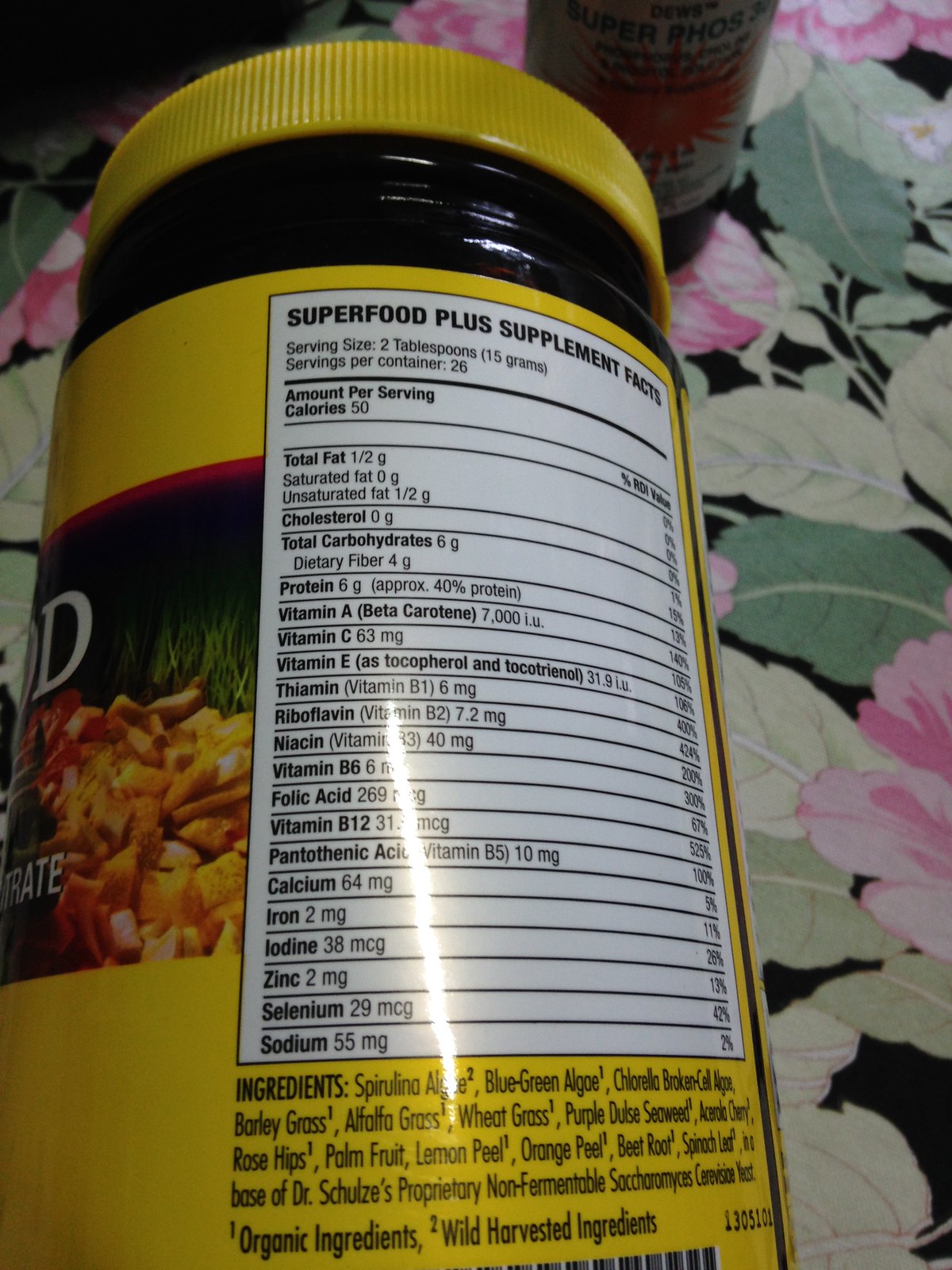This image depicts the nutritional label of the Superfood Plus Supplement shown on the back of a yellow jar with a yellow screw-on lid. The jar, made of dark brown glass to protect its contents from light, is positioned on its side on a flat surface featuring a floral tablecloth with a black background, light and dark green leaves, and pink flowers. Although the resolution is too low to read all details, visible nutritional information includes 1.5g of fat, 6g of protein, and various vitamins and minerals such as vitamins A, C, E, thiamin, riboflavin, vitamin B12, folic acid, iron, and sodium, though their amounts are illegible. The label indicates the serving size is 2 tablespoons with 26 servings per container, and each serving contains 50 calories. On the left side of the label, partially visible text suggests it may recommend refrigeration and displays some indistinct orange pieces, possibly cut-up vegetables or other ingredients.